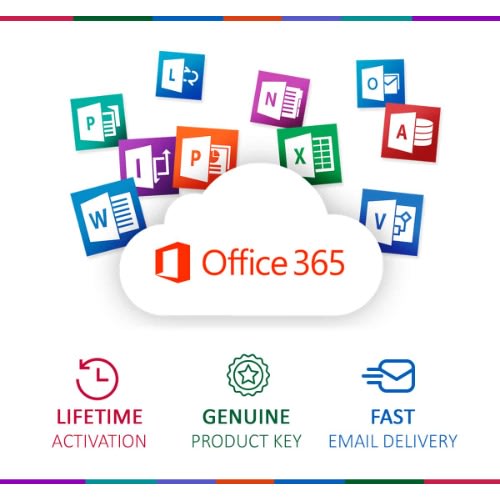This graphic of Microsoft Office 365 prominently features a cloud at the center of a web page, accompanied by the Microsoft Office logo and the name "Office 365" in red text. Behind the central cloud, a series of icons represent various Office programs, including a blue box for Word, a green box for PowerPoint, a green box for Excel, and additional programs indicated by the letters A, O, and L.

Below the central cloud graphic, three distinct icons are displayed. The first icon, colored purple, signifies "Lifetime Activation" and is represented by a clock icon. The second icon, placed centrally and shaped like a medallion with a star, denotes "Genuine Product Key". The third icon is blue and depicts fast email delivery, illustrated by an envelope with dash lines on its left side.

The entire graphic is framed with a multicolored border, featuring a spectrum of hues including purple, red, green, orange, and lilac, adding a vibrant and dynamic touch to the visual representation of Office 365.